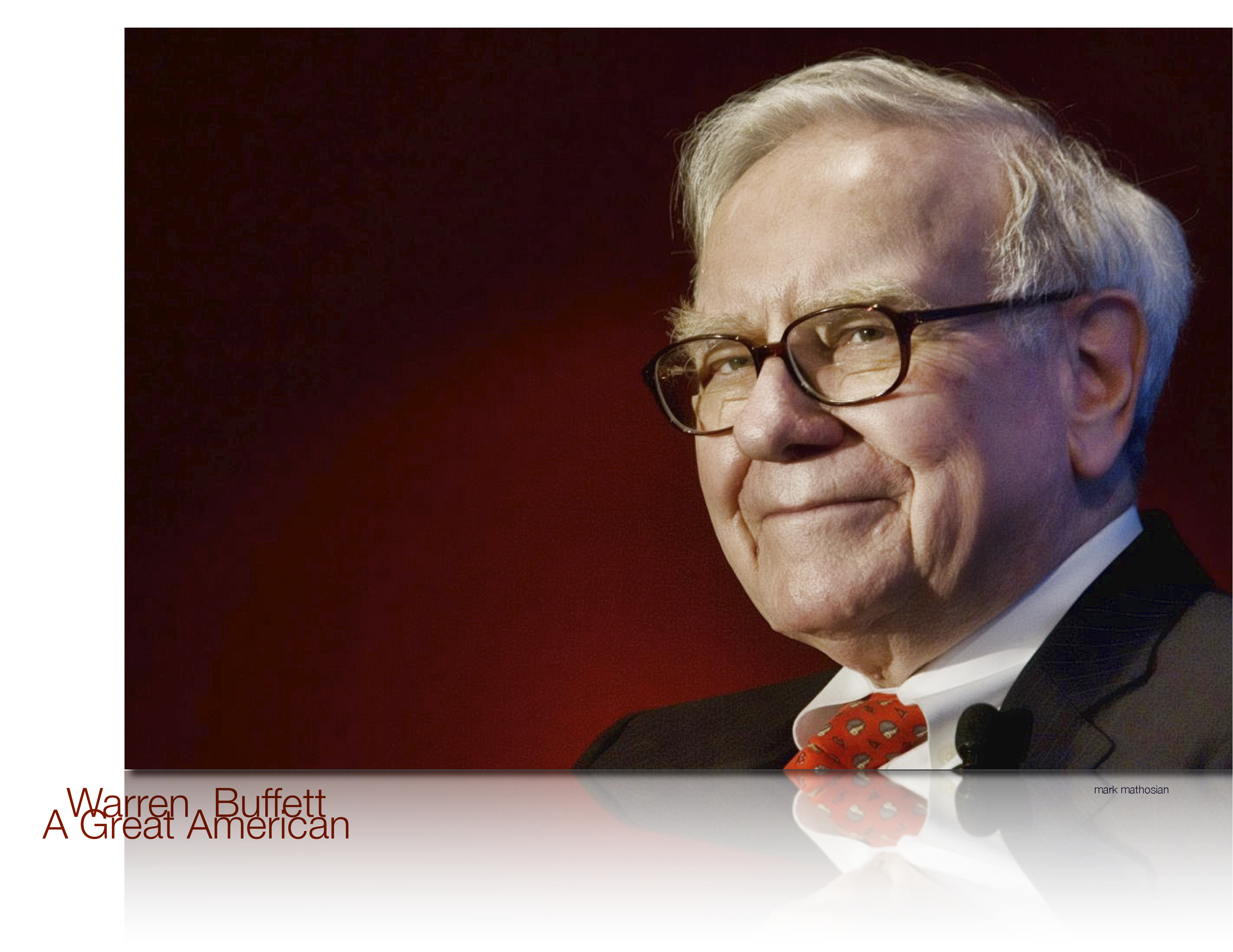The close-up image features an older gentleman, Warren Buffet, identified by text stating "Warren Buffet, a great American" to the left and "Mark Mathosian" in small writing to the right. He has short gray hair styled in a side part and wears black-rimmed glasses that frame his hazel eyes. His expression is warm, characterized by a closed-mouth smile that accentuates the wrinkles around his mouth. His attire includes a black suit jacket paired with a white button-down shirt and a red tie with intricate tan and blue patterns. The background transitions from black at the top to burgundy in the middle, adding depth to the portrait. The reflective surface below the photo captures a mirrored image of his face, tie, and suit jacket, suggesting the photo was taken over a shiny table or the roof of a car.